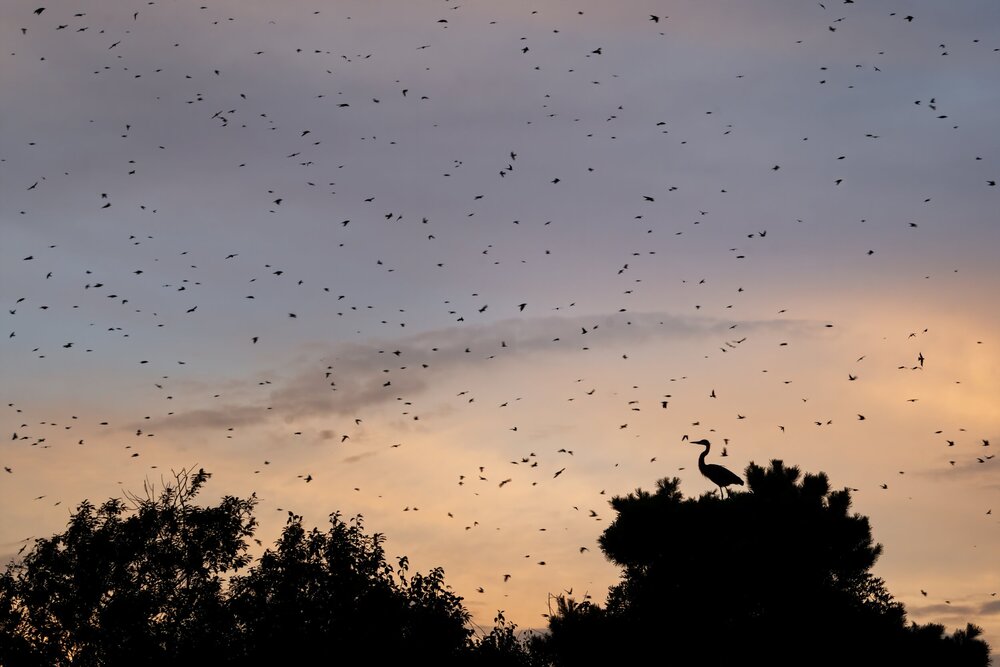This square, full-color photograph captures an outdoor scene at dusk, showcasing a predominantly sky-filled composition with a blend of light blue and light pink hues transitioning to darker shades as the sun sets. Centrally, wisps of clouds add texture to the fading light. Along the bottom edge, silhouettes of trees form a dark boundary, with a notable presence of a large, crane-like bird perched on the top of a tree in the lower right corner. Scattered throughout the sky are numerous indistinct black shapes, likely birds or bats, numbering easily over a hundred, adding dynamic movement to the tranquil evening sky.